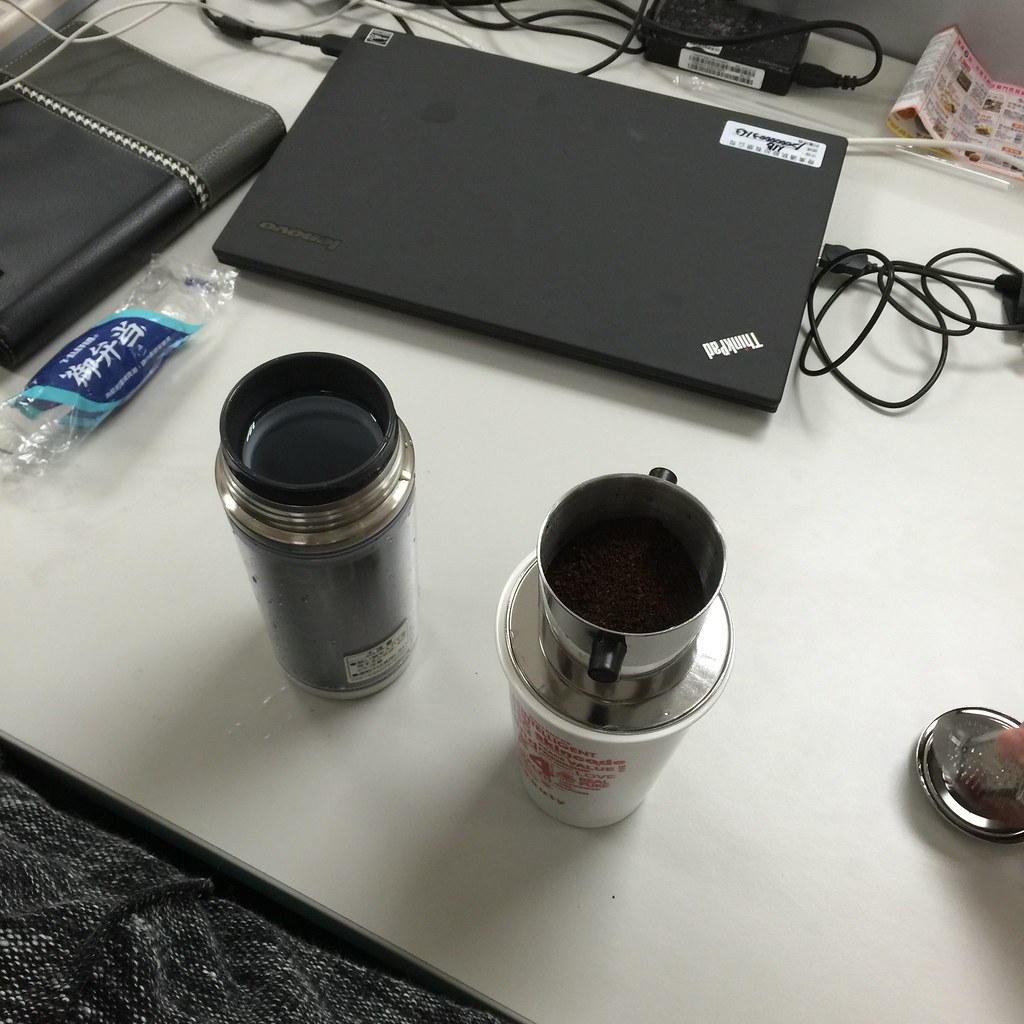The image depicts a cluttered white desk viewed from above. On the desk is a black Lenovo ThinkPad laptop, closed, with wires attached to the side and back. To the left of the laptop is a black leather-bound notebook. Next to the notebook lies a transparent glass mug with a black lid, and a white cup without a lid, which seemingly contains coffee beans or something resembling dirt. To the right of these mugs, a sleek, crystal-clear mouse is visible. Various papers are scattered in the background along with a plastic bag that has Chinese writing on it. In the bottom left-hand corner, there's a gray and white cloth, possibly part of a couch, and in the top right, a menu from a restaurant is partially visible. A finger appears to be touching the metal top of the white cup.